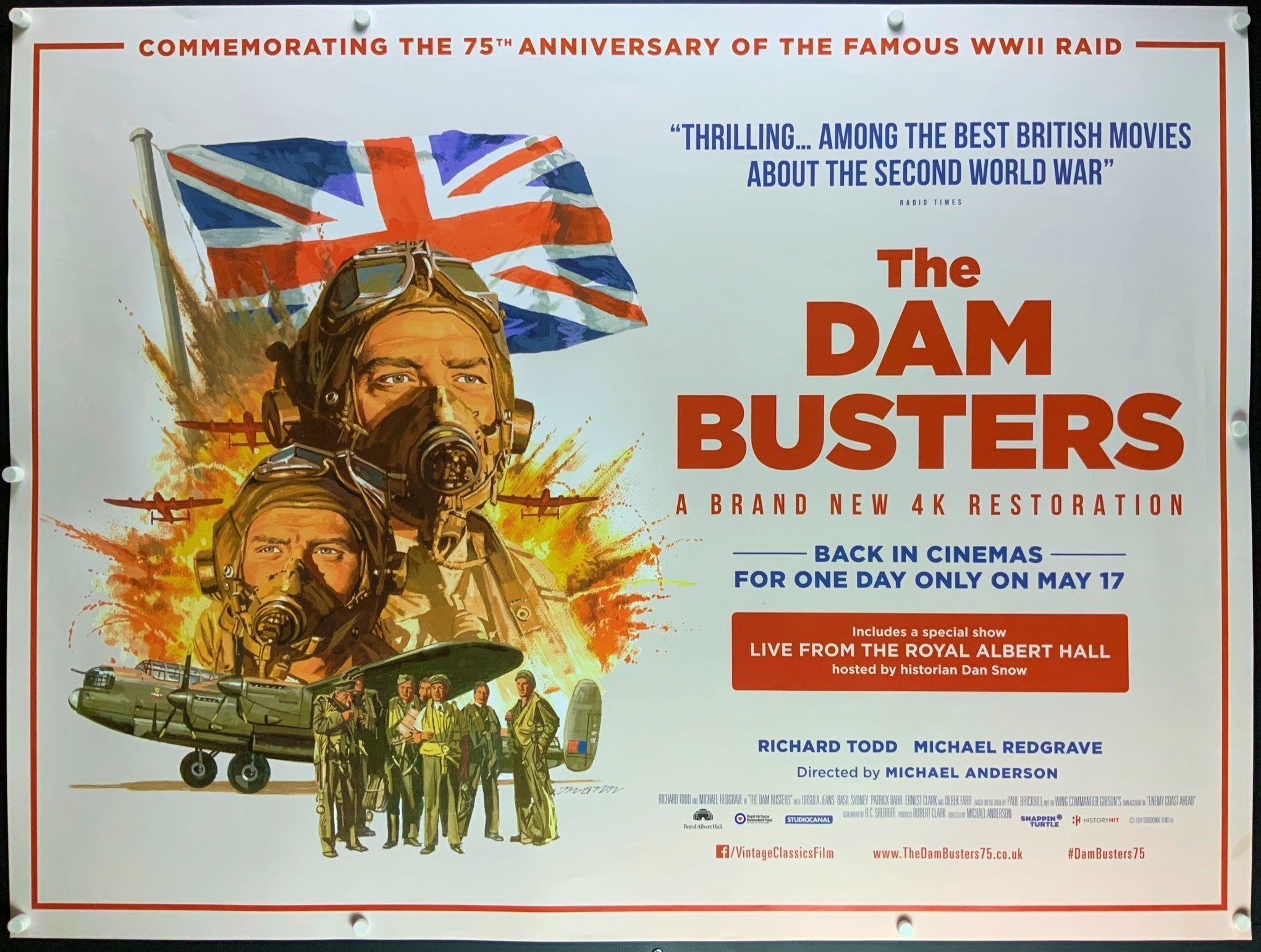This is a detailed promotional poster for the movie "The Dam Busters," commemorating the 75th anniversary of the famous WWII raid. The poster is pinned to a wall with 10 white thumbtacks, two at each corner and additional ones along the sides and top and bottom. The background of the poster is white, bordered by a narrow red band.

At the top, in red letters, the text reads: "Commemorating the 75th anniversary of the famous WWII raid." Below that is an illustration featuring the British Union Jack flag, two large silhouettes of fighter pilots in their gear with air masks and goggles, surrounded by explosions and silhouettes of planes. Underneath this, there's a side profile of an olive-colored fighter plane with several uniformed men, including some pilots with parachutes, standing in front of it.

On the right side, the text in blue letters highlights: "Thrilling, among the best British movies about the Second World War." Following this, in bold red block letters, the title "The Dam Busters" is prominently displayed, along with the note of "A brand new 4K restoration." Below that, in blue, it states: "Back in cinemas for one day only on May 17th."

Continuing, a red rectangle with white text announces: "Includes a special show live from the Royal Albert Hall hosted by historian Dan Snow." Beneath this, the names Richard Todd and Michael Redgrave are listed, followed by the director Michael Anderson. At the very bottom, the text includes "Vintage Classic Films" and additional information like a website URL and a hashtag.